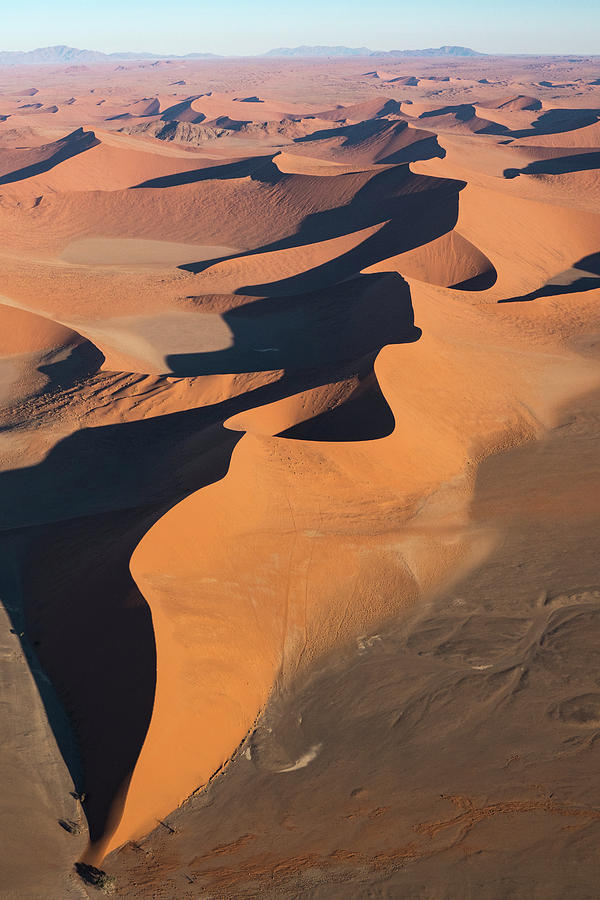The image depicts an expansive desert landscape, assumed to be on Earth or possibly another planet, characterized by a stunning combination of sand dunes and wind-eroded formations. In the very background, a light blue skyline meets a mountainous or hilly region colored in gray. The terrain transitions from these rugged hills into the foreground where sandy flatlands stretch out, sporadically marked with subtle hills etched into the desert floor. The sand varies in hues from yellows, oranges, and browns to nearly black shades, creating diverse shadows and textures across the scene. The surface is dotted with craters and ravines, emphasizing the dynamic interplay of light and shadow. At the forefront, the wind appears to have shifted the sand, revealing deeper layers that appear almost rust-colored.